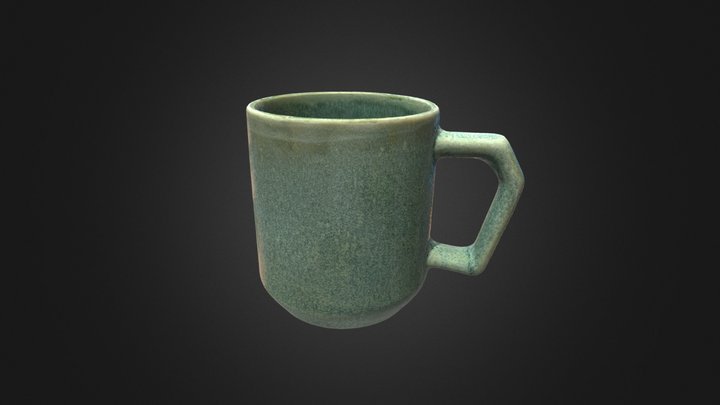The image showcases a teal turquoise mug set against a black background that lightens subtly towards the center. The mug, potentially handmade, features a unique design with black specks scattered throughout its matte finish. Its handle, facing right, is not the typical round shape but rather polygonal with angular edges, almost resembling an ear. The mug tapers down to the base, giving it a slight gradient in shape. The rim of the mug and the interior share a creamier, slightly stained color. The lighting from above highlights reflections on the handle and the rim, adding to its textured appearance. The overall simplicity of the scene emphasizes the detailed craftsmanship of the mug, standing out vividly against the dark backdrop.